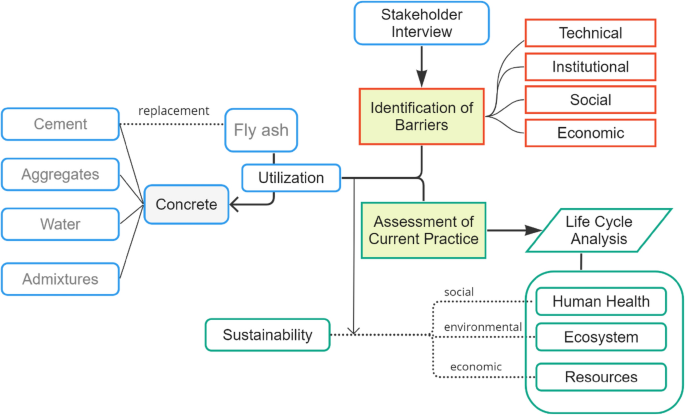This rectangular flowchart diagram, set against a plain white background with no visible borders and dimensions approximately 5 to 6 inches wide and 3 to 4 inches high, details a systematic assessment and workflow related to concrete and sustainability practices. Dominated by various colored boxes and connecting arrows, it visually organizes the process into distinct sections.

At the top center, a white rectangle with beveled edges and a blue outline, labeled "Stakeholder Interview," serves as the starting point. Below this, an arrow directs to another rectangle labeled "Identification of Barriers," flanked by four red boxes to the right indicating specific barriers: Technical, Institutional, Social, and Economic.

Progressing downward, the flowchart points to "Assessment of Current Practices." From here, arrows extend to various elements on the right, such as a green-outlined box labeled "Life Cycle Analysis," encompassing aspects like Human Health, Ecosystems, and Resources. Adjacent to this are areas focused on Social, Environmental, and Economic factors, connected by lines demonstrating their interrelation.

To the left of "Assessment of Current Practices," additional lines link to "Utilization," which branches upwards to "Fly Ash" and downwards to "Concrete." Further extending leftward, it denotes materials involved: Cement, Aggregates, Water, and Admixtures—all essential components in concrete formation.

The use of color—green, gray, black, red, and blue—enhances the differentiation of categories and connections, illustrating a comprehensive flowchart typical of those used in scientific or industrial contexts to map out processes and assessments systematically.